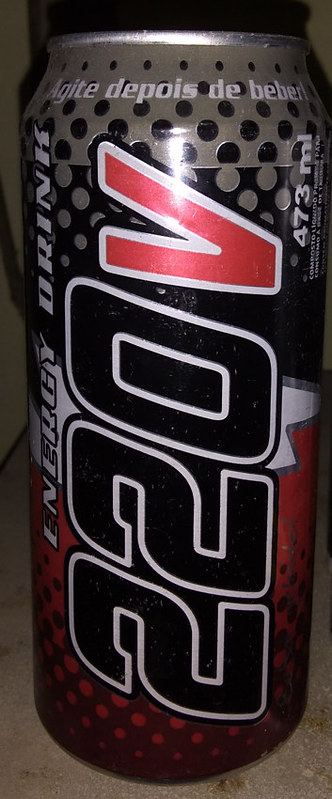This close-up photograph showcases an aluminum energy drink can positioned on a granite kitchen counter. The image, tightly cropped to the dimensions of the can, emphasizes its tall, rectangular shape while the bright lighting highlights the can's details, leaving the background obscured. The can's design features a dominant gray color at the top, transitioning to black dotted with large gray bubbles, which resemble the halftone effect. The can displays prominent, vertical text "220V" in black and "473ML" in white. Encircling the top edge, in white lettering, it reads "Agite depois de beber,” which is Portuguese for "Shake before drinking." This text is bordered with black outlines, reminiscent of Impact font often seen in meme text. The bottom section of the can is maroon, adorned with pink and maroon bubbles. Diagonally on the left, in white letters, it states "energy drink," while a large red "V" with a white outline stands out, contributing to the dynamic, eye-catching design of the can.